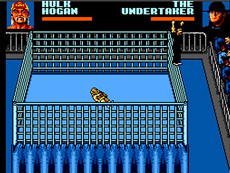A nostalgic screenshot from an 80s-style video game depicting a classic wrestling match. The scene is set in a blue boxing ring, dominating the center of the image. In the upper left corner is a pixelated portrait of a blonde man with a red bandana, identified by the accompanying text as Hulk Hogan, the iconic wrestler. To the right of the ring, another pixelated image shows a man wearing a black hat, labeled as The Undertaker, a formidable opponent known in wrestling lore. In the ring, Hulk Hogan lies sprawled on his back, seemingly defeated, while The Undertaker stands triumphantly on the ring's edge. The background reveals a sparsely detailed audience, their figures barely visible but clearly engrossed in the unfolding drama. Surrounding the entire scene is a gray border, framing this vintage wrestling bout.